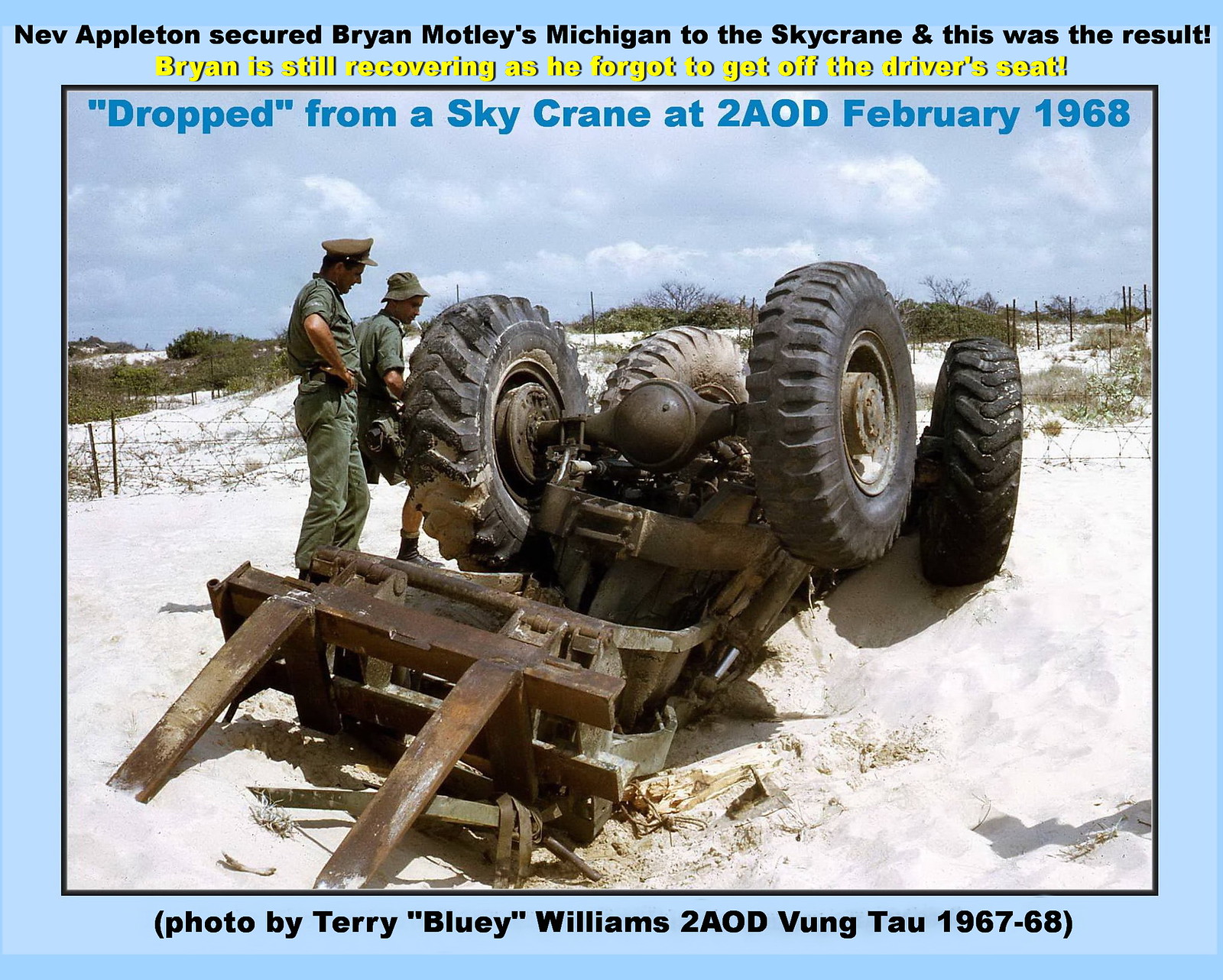The framed photograph, bordered in light blue, depicts a military scene likely from the Vietnam War. It shows a large vehicle flipped upside down on a sandy beach-like area with dunes and grass in the background. The vehicle, which appears to have been a part of a mishap involving a sky crane, is surrounded by two soldiers in dark forest green uniforms, one working on the vehicle and the other supervising. The top of the photograph features black text stating, "Nev Appleton secured Brian Motley's Michigan to the sky crane and this was the result. Brian is still recovering as he forgot to get off the driver's seat." Additionally, in bright yellow text, it notes, "Dropped from a Sky Crane at 2AOD, February 1968." Below the photo, a caption reads, "Photo by Terry 'Bluey' Williams, 2AOD, Vung Tau, 1967-68."